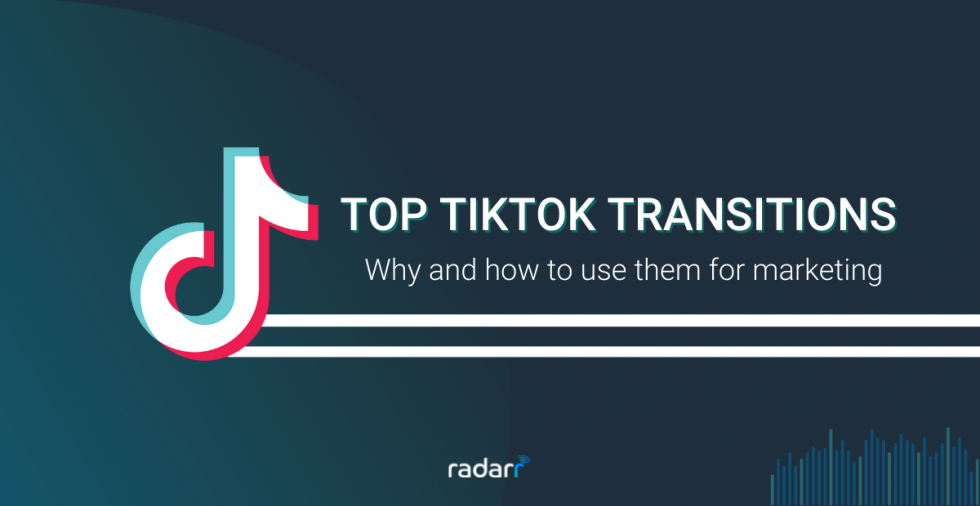The image is a wide rectangle, approximately twice as wide as it is tall, featuring a dual-toned background that transitions from an aquamarine hue on the left to a dark blue, almost black, shade on the right. Dominating the center of the image is the TikTok logo, a stylized red, white, and blue "D" shaped like a musical note. This emblem is the most prominent element, occupying roughly one-third of the image's vertical space and a fifth of its horizontal space. The circular part of the note doesn’t close fully towards the middle.

Beneath the TikTok logo, spanning the width of the image, are two thick, white horizontal lines extending from the logo to the right edge. Above these lines, white text in all capital letters reads "TOP TIKTOK TRANSITIONS." Below this, smaller white text in sentence case states "Why and How to Use Them for Marketing," with only the first word capitalized.

At the very bottom of the image, centered, is the word "radar" in lowercase white letters, followed by a blue arrow pointing to the right. In the lower right corner, a series of thin vertical bars—resembling a volume bar graph—are displayed in shades of blue and pale green against the dark background. These bars, numbering around 20 to 30, fill the lower right quadrant of the image, contributing to its dynamic visual composition.